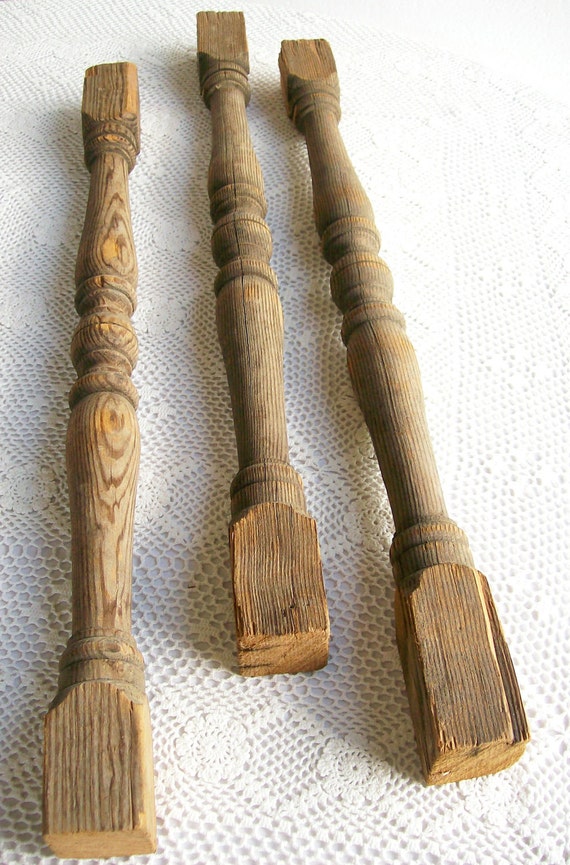The photograph showcases three intricately crafted wooden objects, likely table legs or banisters, lying parallel on a cream-colored crocheted tablecloth with an ornate lace design, featuring delicate flower patterns. Each wooden piece is unpainted, revealing a distinctive wood grain and cylindrical design, with rectangular sections at both the top and bottom. The photograph is well-lit, highlighting the natural wood texture and the meticulous craftsmanship of the pieces, which exhibit both straight and curved patterns. The legs are arranged with the one on the left positioned slightly lower, the middle one above the others, and the third aligned more closely with the first, all set against the backdrop of a finely detailed white fabric.